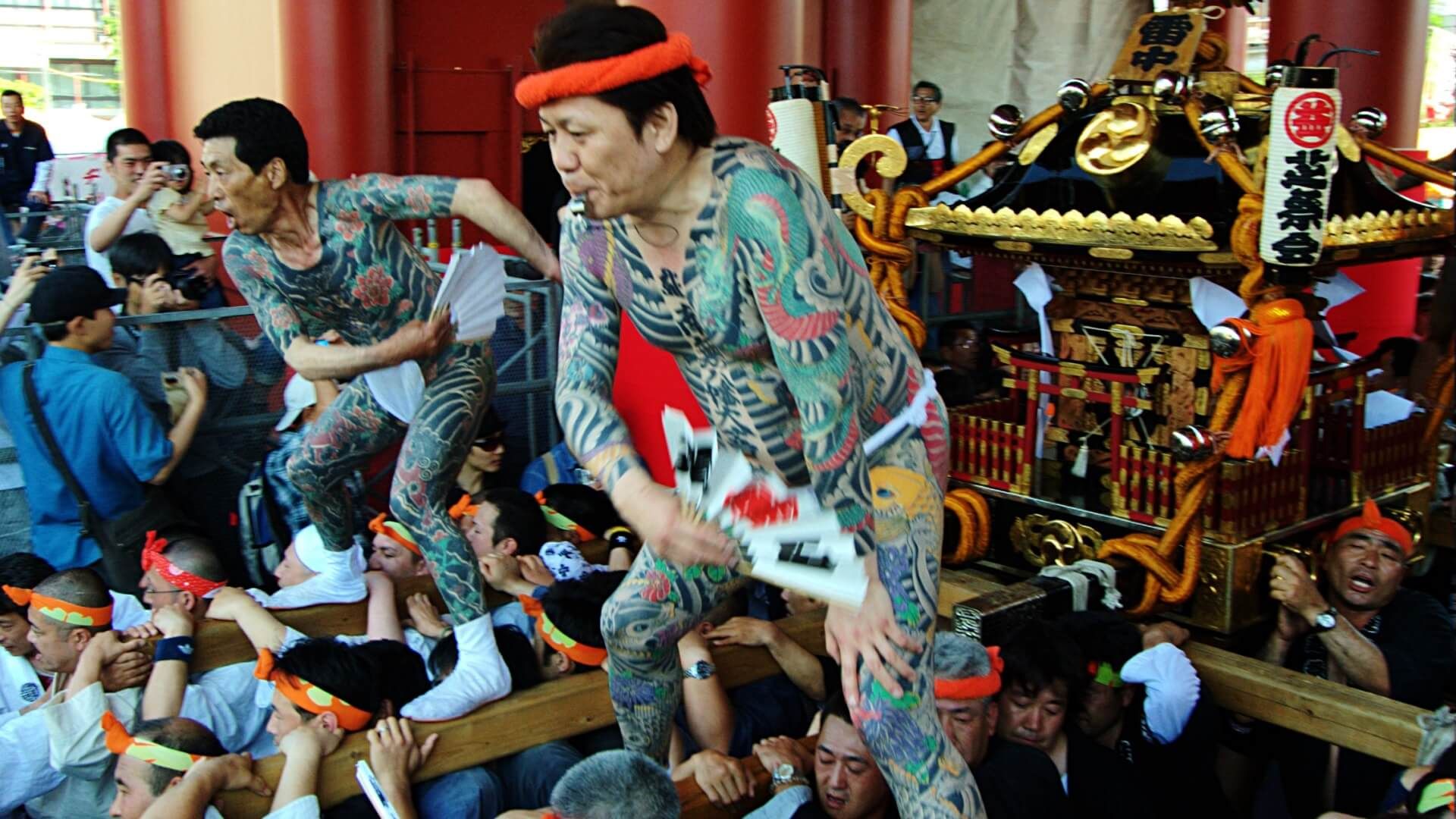The image features two heavily tattooed men standing atop a raised platform supported by numerous individuals below. Each man stands with one foot on a wooden beam, and they are minimally dressed in white loincloths. The men on top hold oriental fans, with one of them wearing a red headband and blowing a whistle. The group below them, also wearing headbands, is lifting the platform which functions as part of a colorful, antique-looking parade float. This float, adorned with red, gold, and black colors, lanterns, and text, gives off a strong Asian aesthetic akin to a traditional dojo or ceremonial procession. In the background, a crowd gathers, with a few onlookers capturing the event with their cameras, indicating that this is part of a vibrant, ceremonial parade or demonstration.